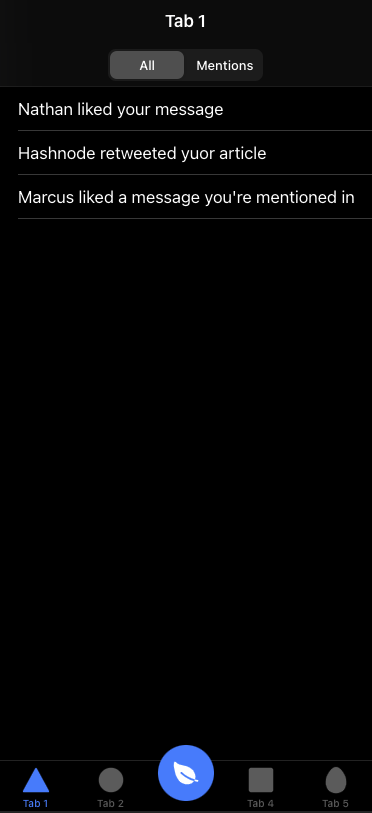The image depicts a vertically-oriented rectangular box set against a completely black background. At the very top center of the box, the label "Tab 1" is displayed in white lettering. Below this title, there are options to select either "All" or "Mentions," with "All" currently highlighted. 

Further down, several lines of white text convey the following notifications:
1. "Nathan liked your message."
2. "Hashnode retweeted your article," with the word "your" misspelled as "yuor."
3. "Marcus liked a message you're mentioned in."

The lower half of the screen features a considerable amount of blank space up until the very bottom, where several navigation elements are present. These elements include:
- A bright blue triangle labeled "Tab 1," also in bright blue.
- A gray circle labeled "Tab 2."
- A bright blue circle centered with a white leaf symbol.
- A gray square labeled "Tab 4."
- A gray, rounded teardrop shape labeled "Tab 5."

The overall layout suggests an interface with multiple tabs and notifications, designed with a clean, minimalist aesthetic.